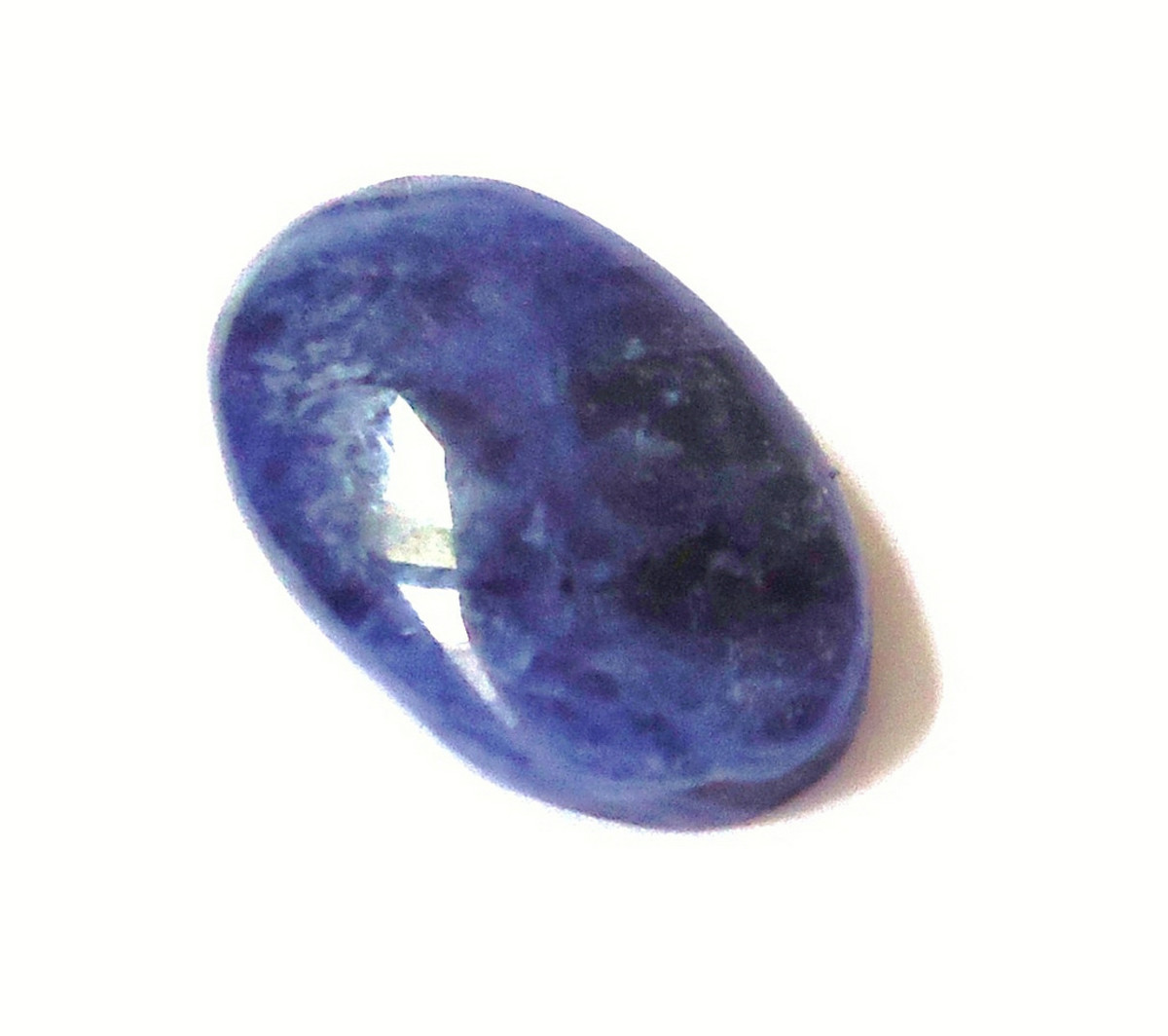This image showcases a polished, oval-shaped gemstone or precious stone, predominantly featuring a marbled mix of royal blue and black hues with lighter blue and white speckles. The stone, angled roughly at 45 degrees, is centrally positioned on a white background, which appears to be either a white countertop or a photo backdrop. The resolution of the image is somewhat low, giving it a slight fuzziness, as if it were highly zoomed in. The polished surface of the stone casts a light gray, tan-tinged shadow on the lower right-hand side. Additionally, there's a reflection on the stone's left side, where a white, hockey stick-shaped glare indicates it was taken in a bright room during daylight, possibly near a window given the faint silhouette of trees and sky in the background. The image is free of any text, focusing solely on the smooth and shiny multi-colored gemstone which might be part of a rock collection.